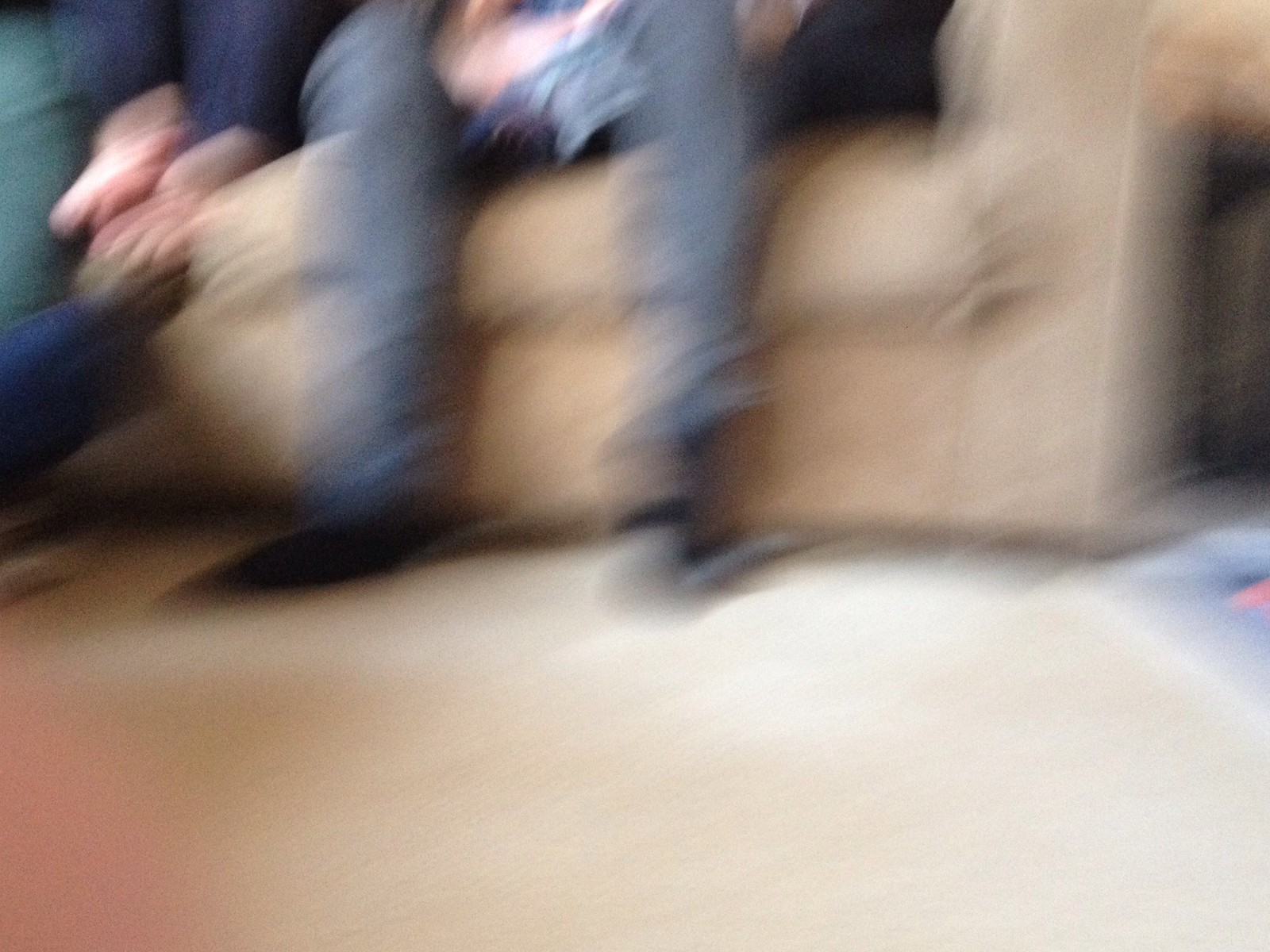This is a very blurry image depicting a tan couch with at least two people seated on it. The first person, wearing gray pants and black shoes, appears to be sitting with their hands on their lap. There is a flesh-colored object or possibly their hands resting on their lap. A black pillow is visible on the couch next to them. The second person on the couch seems to have bare feet, which are propped up on the couch. A teal-colored item is positioned next to this person, though it is unclear if it is another person or an object. Additionally, there is something blue beneath where the second person's feet rest, possibly indicating someone sitting on the floor. The overall scene is intentionally blurred, making specific details difficult to discern. The floor is tan, and there are various objects scattered, including something black to the right and pink and blue items on the floor.